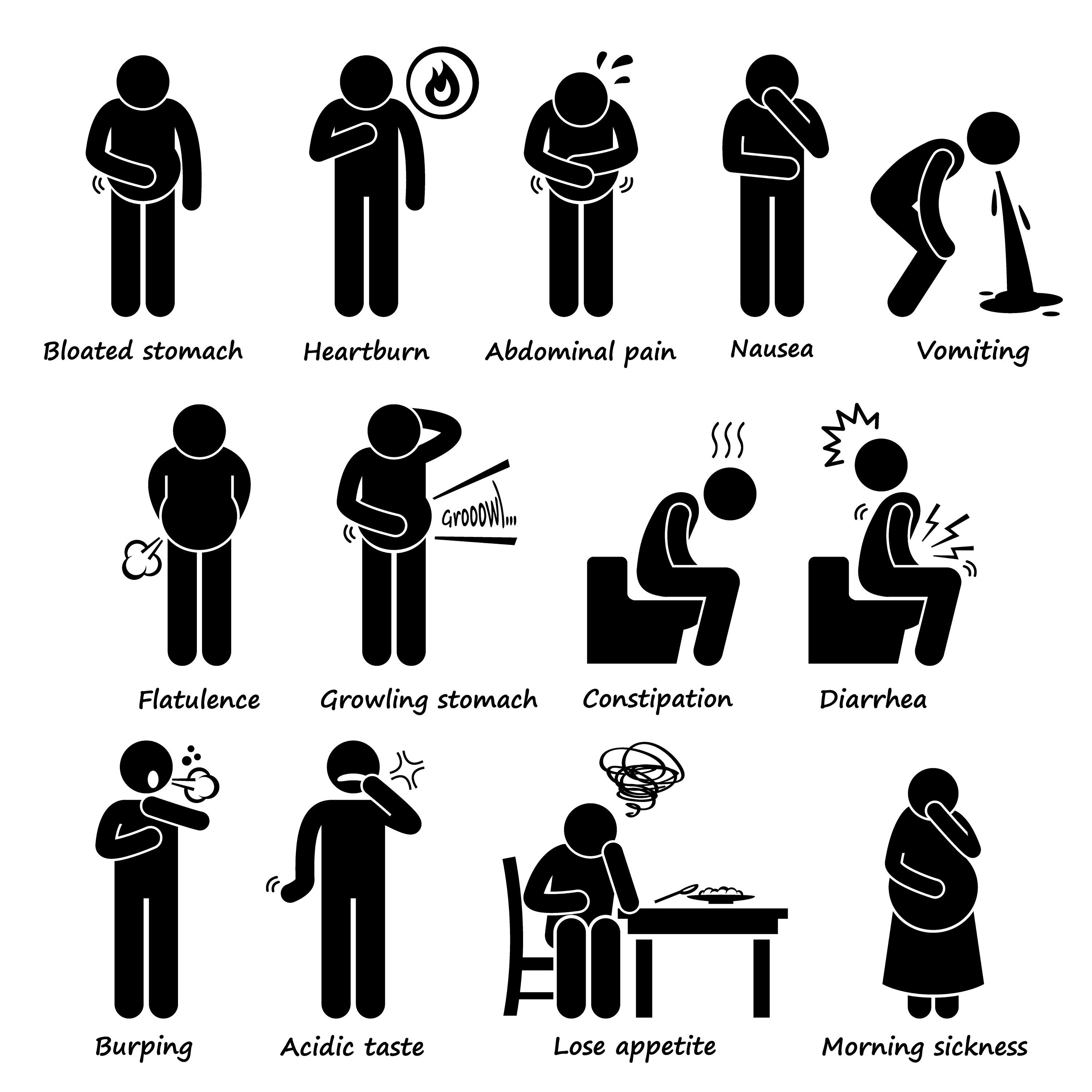The illustration is a black and white infographic featuring a series of simplistic, faceless stick figures, each representing a different symptom of various sicknesses. At the top left, a figure clutching its stomach indicates a "bloated stomach." Next, a figure holding its heart with a fire icon beside it symbolizes "heartburn." The central top row includes a figure double-arming its abdomen for "abdominal pain," one looking nauseous about to vomit for "nausea," and another ejecting vomit for "vomiting."

Moving to the middle row, the first figure has a cloud near its butt representing "flatulence," followed by a figure with a growling sound effect for "growling stomach," a hunched figure for "constipation," and then one depicting "diarrhea" with indications of ejecting waste. The bottom row begins with a figure burping, marked by a gas symbol near its mouth for "burping," followed by "acidic taste" portrayed by a figure with a grimacing expression. Next is a figure sitting at a table with untouched food labeled "loss of appetite," and finally, a pregnant figure indicating "morning sickness."

Each stick figure is positioned in unique stances to represent their respective symptoms, with corresponding descriptive text beneath, making the infographic a clear and detailed depiction of various health issues.